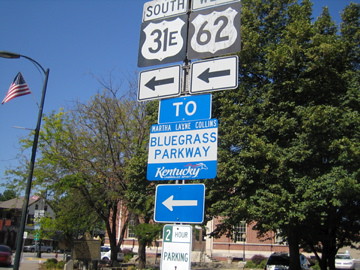This image features an extensively detailed traffic sign positioned at an intersection. The sign includes multiple directives: at the bottom, there is a "Two-Hour Parking" notice. Above it, a blue directional sign instructs left-bound traffic towards Bluegrass Parkway, indicating the location is in Kentucky. Additional signage directs drivers with two arrows pointing to the left: one for US Highway 31 East (southbound) and another for US Highway 62 (westbound), both guiding traffic in the same direction. The backdrop features a couple of trees and a sizable brick building, possibly a school. On a light pole adjacent to the road, a US flag is prominently displayed, enhancing the scene's quintessentially American atmosphere. There is no visible school zone sign in the vicinity.